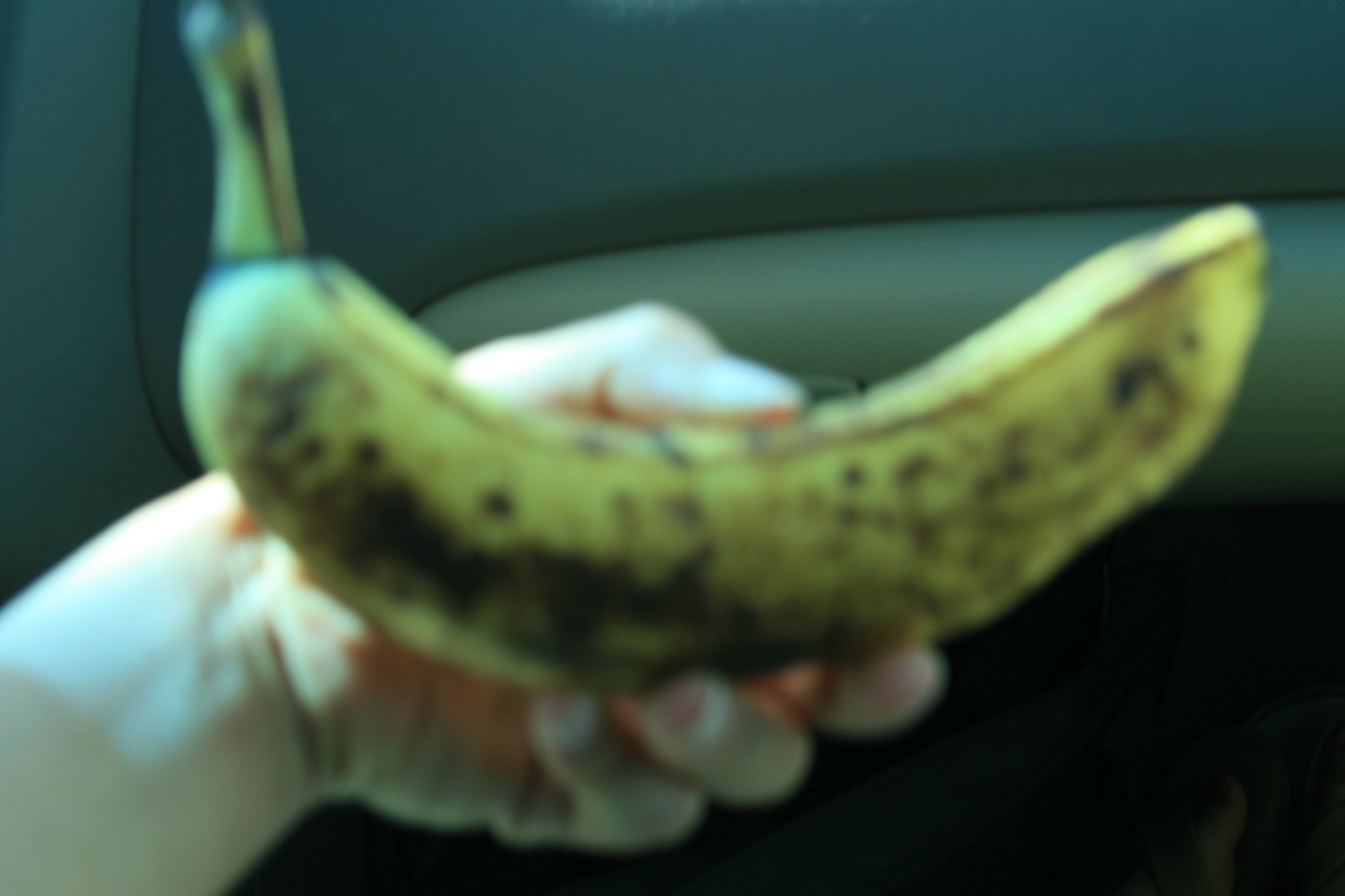This photograph captures a hand holding an overripe banana, rendered in a very blurred and low-quality image. The hand, with light skin and short, clean fingernails, emerges from the left bottom corner of the frame, clasping the banana upright between its thumb and fingers. The banana, positioned horizontally, exhibits a yellow background marred by numerous browned areas and specks, indicative of its overripe state. Its stem remains attached, although it is black around the base. The scene is set in what appears to be the interior of a car, with the glove box and molded plastic dashboard visible behind the hand. The dark, unlit area below, possibly the wheel well or footwell, further contextualizes the setting. The banana itself measures approximately six to seven inches in length, suggesting it is quite large.